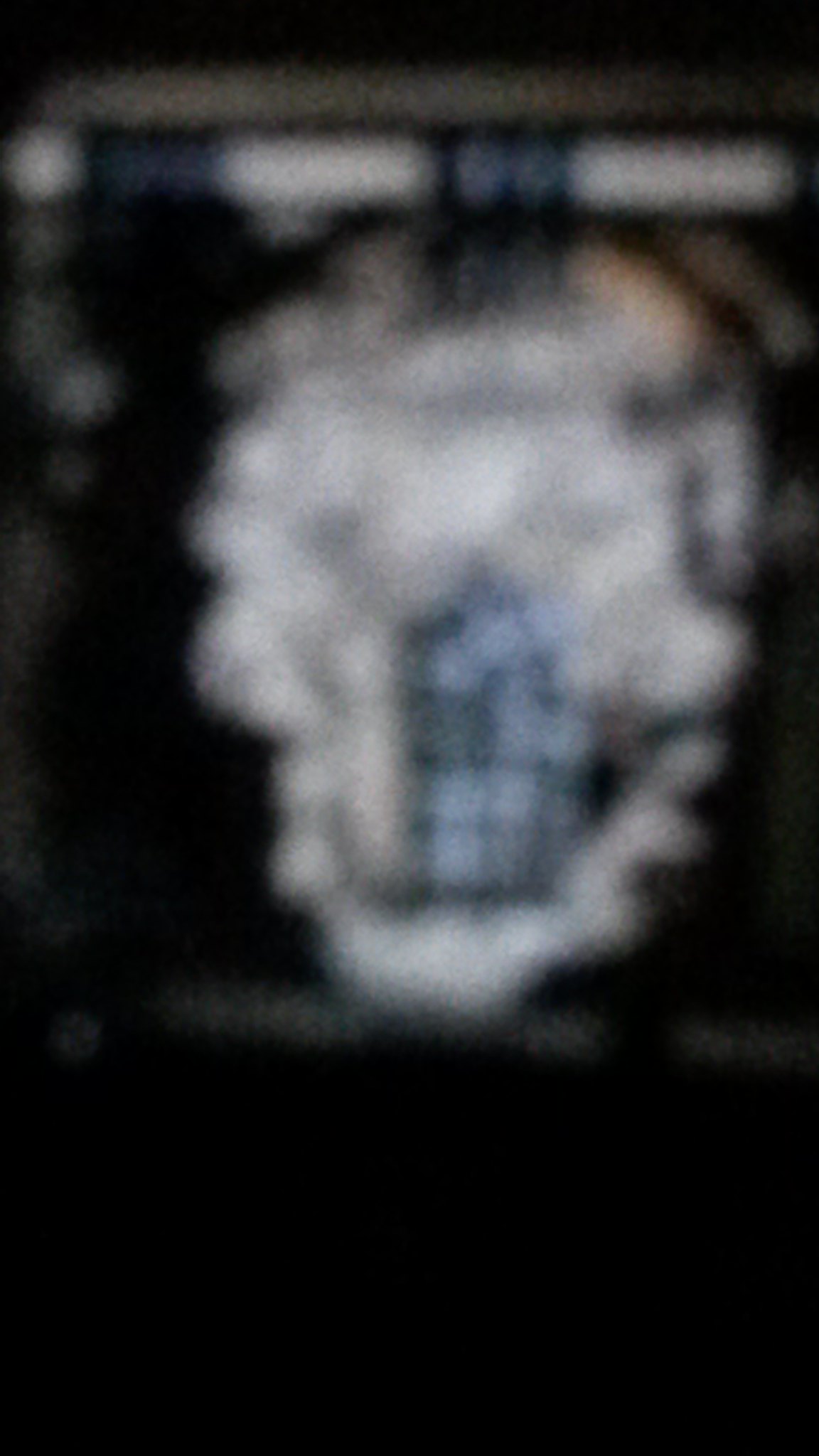The image is extremely blurry, taken at night with a predominantly black background. In the center, there appears to be a white, cloud-like shape, potentially caused by a flash. Surrounding this central shape are storm-like clouds. At the top of this cloudy formation, there's an orange hue reminiscent of Cheetos. The middle section of the image contains a window-like structure with blue and gray checkered patterns, resembling either a skull or a dog with eyes and a mouth. This window or door-like feature is highlighted by various shades of light, including blue, white, brown, and tan. There are horizontal lines with patterns, possibly text or numbers, both at the top and the bottom of the image, adding to the overall complex yet indistinct composition.